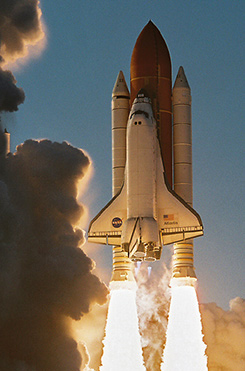This detailed image captures the dramatic moment of a space shuttle launch in a grainy, possibly decades-old photograph. The shuttle, identifiable by its prominent NASA logo on the left wing and the American flag on the right wing, is seen with all its stages intact, indicating it has just taken off. The sky, a medium blue possibly suggesting a time near sunset or sunrise, provides a vivid backdrop to the scene. The massive orange fuel tank and the two white, crayon-like solid rocket boosters are clearly visible. From the bottom of the shuttle, bright, intense yellow flames and a clean jet stream of thrust erupt, generating thick, billowing gray clouds of smoke that envelop the lower part of the image. The focus on the shuttle and the proximity to the ground enhance the powerful and awe-inspiring nature of the launch.